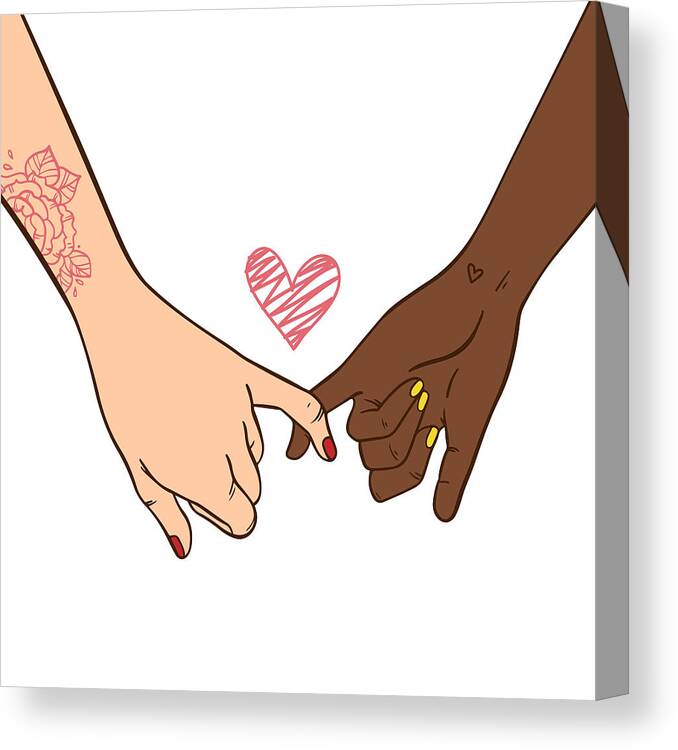The image is a detailed piece of color canvas wall art set against a white backdrop. It features two hands linked by their pinkies, centered on a white background. The left hand, belonging to a light-skinned individual, displays red-painted nails and a partial tattoo of a red rose with leaves just below the wrist. The right hand, belonging to a dark-skinned individual, has yellow-painted nails and a small heart tattoo on the underside of the wrist. Above their interlocked pinkies, there is a red heart with pink scribbles inside it. An interesting aspect of the canvas is that the image isn't confined to the front surface; the dark-skinned arm's image wraps around to the side of the canvas, creating a continuous visual effect. The artwork cleverly utilizes the frame, extending elements of the picture onto the sides, enhancing its overall appearance.